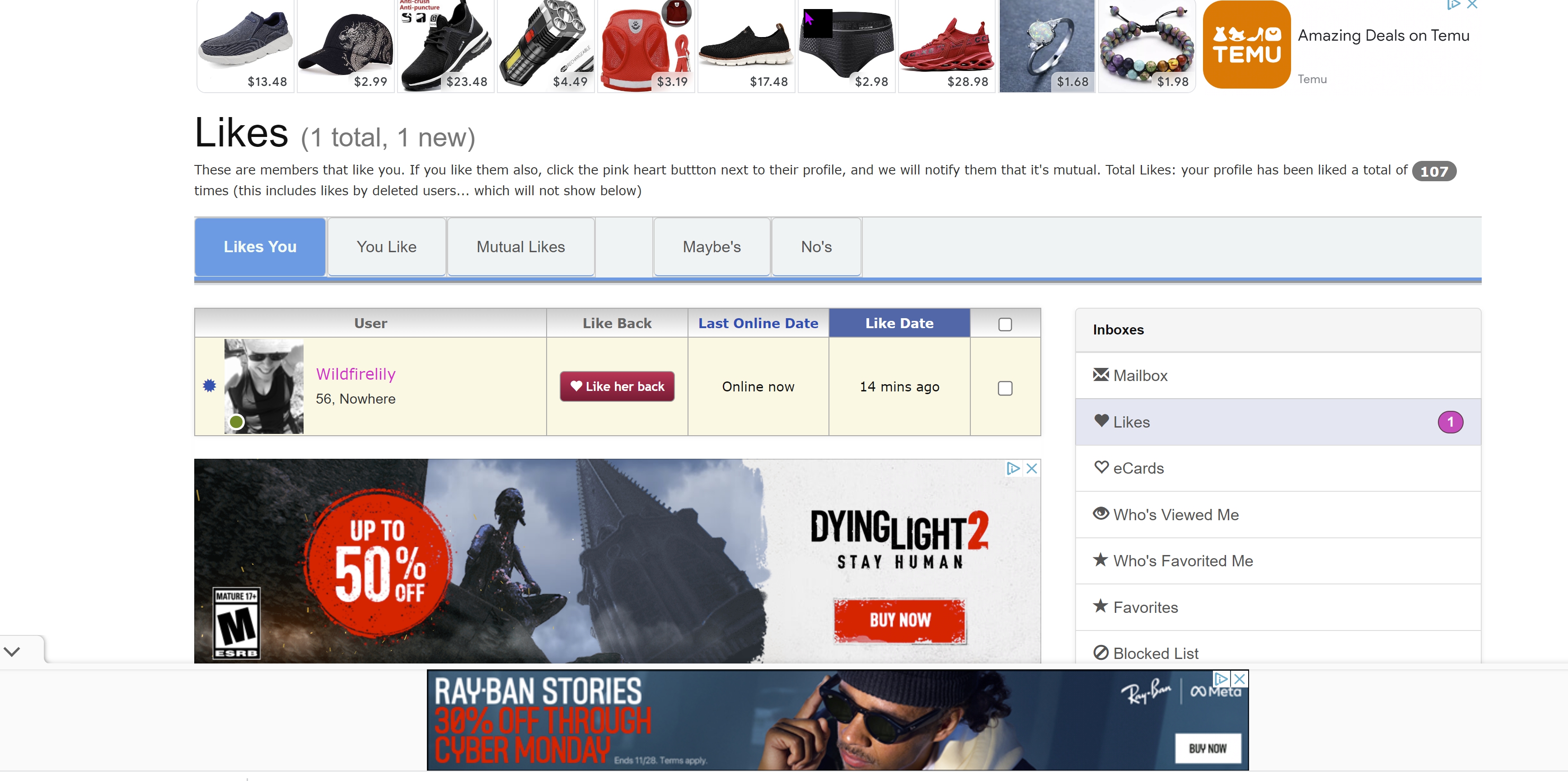The image features a vibrant and detailed webpage showcasing various elements and advertisements related to the brand Tame. 

At the top of the page is a prominent advertisement by Tame, highlighted by an orange icon with "Tame" written in white. The advertisement announces "amazing deals on Tame and their products." Alongside this, a variety of products are displayed with their respective prices: 
- Shoe for $13.48
- Crib for $2.99
- Another shoe for $23.48
- Flashlight for $4.49
- Vest for $3.19
- Yet another shoe for $17.48
- Underwear for $2.98
- A red shoe for $28.99
- Ring for $1.68
- Bracelet for $1.98

At the bottom of the webpage, stats reveal user engagement metrics: “likes, one total, one new.” It instructs users that if they like someone back, they can click the pink heart button next to their profile to notify them that the feeling is mutual. It states that the profile has been liked a total of 107 times, including by users who have since deleted their profiles. This section also displays a profile page with various interaction tabs such as "likes you," "you like," "mutual likes," "maybes," and "no's." The background of this page is grey, while the highlighted tab, “likes you,” is blue.

Below this, the user "WhitefireLily56Norway" is shown as online, with options to "Like her back" via a red button, and information that she was last online 14 minutes ago. The right side of the page features additional navigation options, including inboxes, mailbox, likes, e-cards, "who viewed me," "who favorites me," and "favorite blog list." A pink icon signifies that one user has liked the profile.

The bottom section of the page includes multiple advertisements: one for "Dying Light 2: Stay Human" on the bottom-left corner and another for "Rape and Stories" offering "30% off through Cyber Monday," with the text in red.